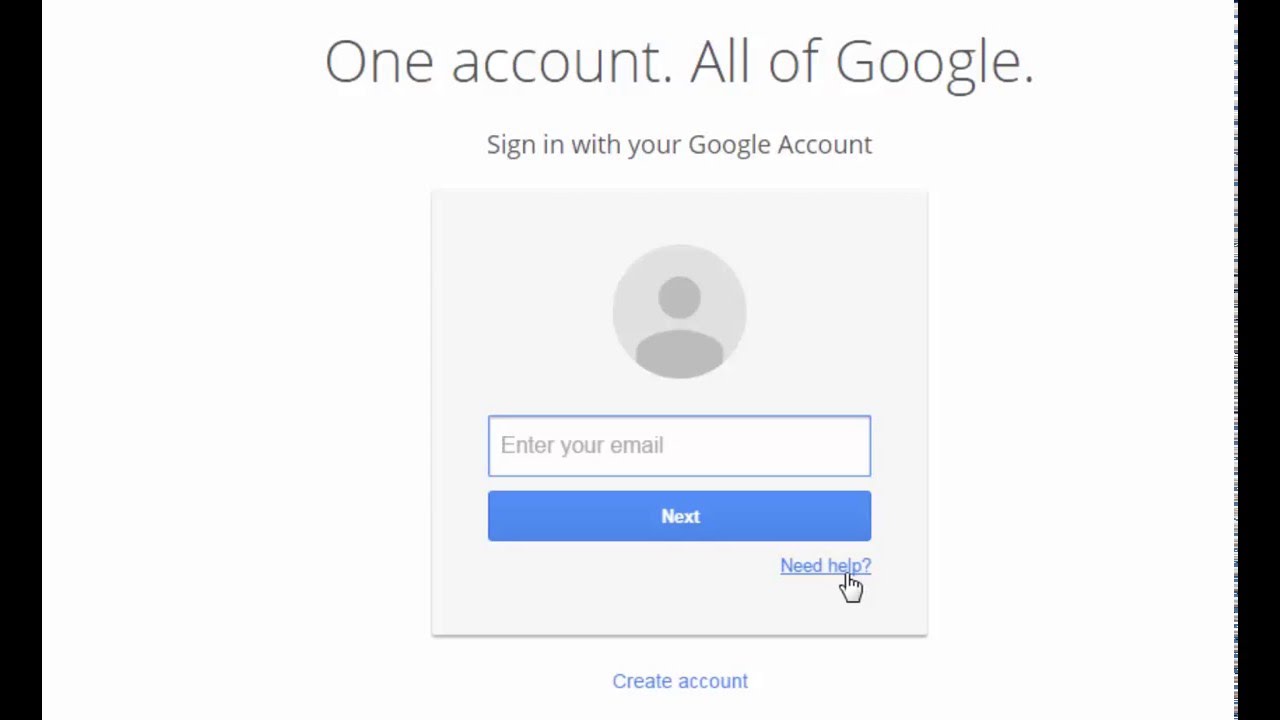This image depicts a Google account login page against a white background. At the top of the page, the text "One account. All of Google." is prominently displayed in black, followed by the instruction "Sign in with your Google Account" also in black text. 

Centrally positioned, there is a light gray square containing the login elements. The square features a profile icon that is a combination of gray and dark gray, with the dark gray portion representing the silhouette of a person's face and upper body.

Beneath the profile icon, there is a white text box outlined in blue with the placeholder text "Enter email" written in gray. Below this text box is a blue button with the word "Next" written in white.

To the bottom right of the "Next" button, the blue and underlined text "Need help?" is visible, with a white mouse cursor, outlined in black and shaped like a hand, pointing to it.

At the very bottom of the image, the text "Create account" appears in blue, indicating the option for users to create a new account if they do not already have one. The overall design is clean and intuitive, guiding users seamlessly through the sign-in process.